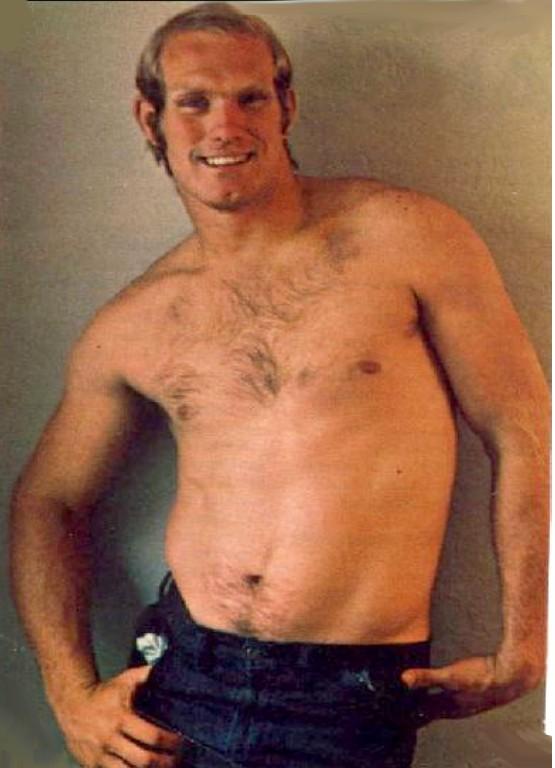This is a vintage photo of Terry Bradshaw, the iconic football player, taken during the 1970s era. He appears shirtless and is dressed in dark blue jeans, with his right thumb hooked into the pocket, slightly pulling it down, revealing a bit of the pocket's light-colored interior. Bradshaw’s pose is casual and confident, with his left arm resting on his hip and his body slightly twisted, leaning back against a wall that has an ambiguous color – possibly gray, eggshell yellow, or beige – with a shadow creating a soft effect. His face is adorned with chin stubble, and he sports sideburns alongside his short blonde hair, which is noticeably beginning to thin at the top. He has a relaxed smile, showing his ease in front of the camera. His chest has a moderate amount of hair, extending down towards his navel, but his abdomen remains relatively hairless. The lighting in the photograph seems to be centered on his midsection, highlighting his form against the indoor setting.